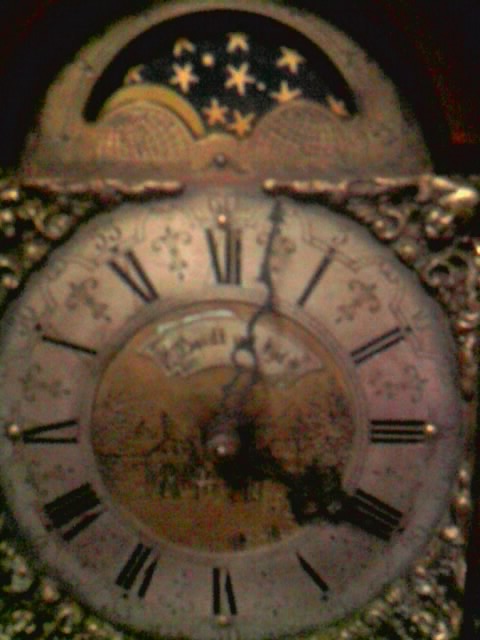This image portrays an ornate clock with a square-shaped top, framed in gold, and adorned with intricate gold etchings, including swirl designs and cherubic figurines in each corner. The clock's face is round and white, accentuated by black Roman numerals and fleur-de-lis motifs between the numbers. The clock hands are black, and the center of the face is gold with a blurred banner and floral scene. Above the clock face, there is a half-circle arch in blue, dotted with yellow stars, likely representing a nighttime scene. The design is intricate, featuring additional decorative patterns in each corner.